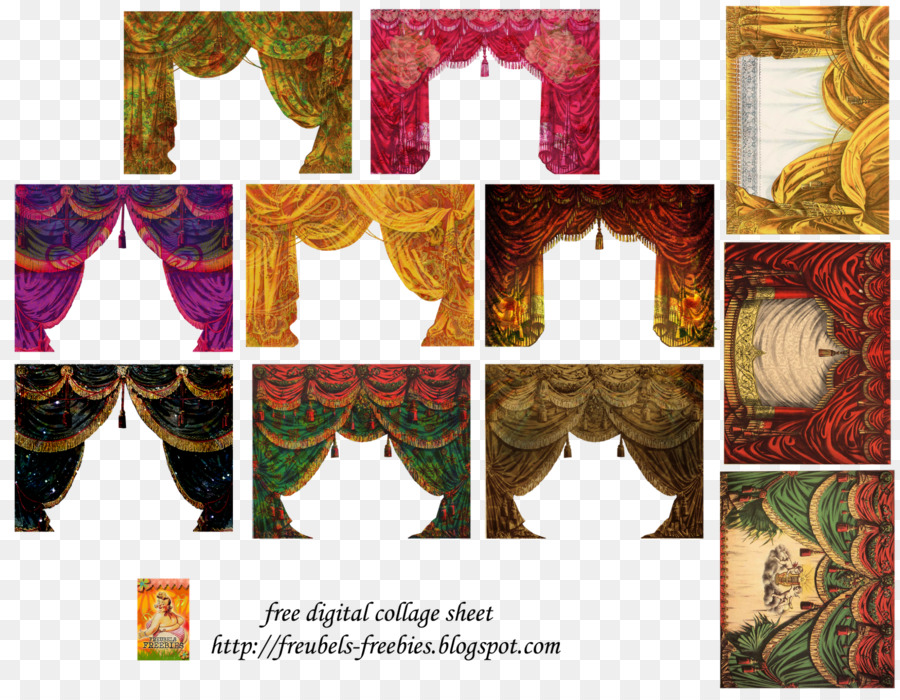The image showcases an ornate and colorful collection of eleven digital curtains arranged against a checkerboard background. The curtains are silken and resemble those used on a theatrical stage, exuding an animated, almost surreal vibe. They are meticulously grouped, with two curtains on the top row, three on the next, three more below that, and an additional three positioned vertically on the right side, rotated by 90 degrees. The colors are diverse and vibrant, including hues of purple, pink, magenta, gold, yellow, black, dark red, green, orange, and brown, with some curtains featuring intricate floral patterns. Beneath the array of curtains, text reads "Free digital collage sheet" followed by a URL: http://freubels-frebies.blogspot.com, along with a small logo of the Freubel’s Freebies blogspot. This image appears to be a digital offering for creative use, likely in PNG format, enabling easy incorporation into various artistic projects.